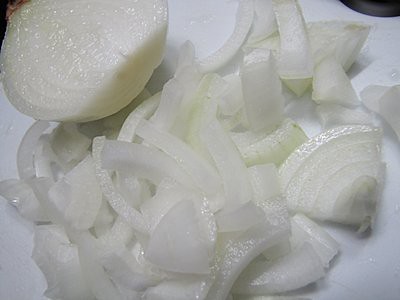This color photograph, taken inside a kitchen with overhead lighting, captures the process of slicing a white onion on a white chopping board. In the top left corner, a half onion rests on its curved side with the flat side facing up. This onion half has had its ends removed and is peeled, displaying a glossy, pearly texture that almost appears wet under the light. To the right, the other half of the onion has been roughly chopped into quarter-sized slices and scattered across the board. The white hues of the onion and chopping board dominate the image, creating a monochromatic effect with subtle shadows adding depth. A tiny bit of a black object, potentially the edge of a frying pan, is visible in the top right corner, providing a hint of the kitchen setting.